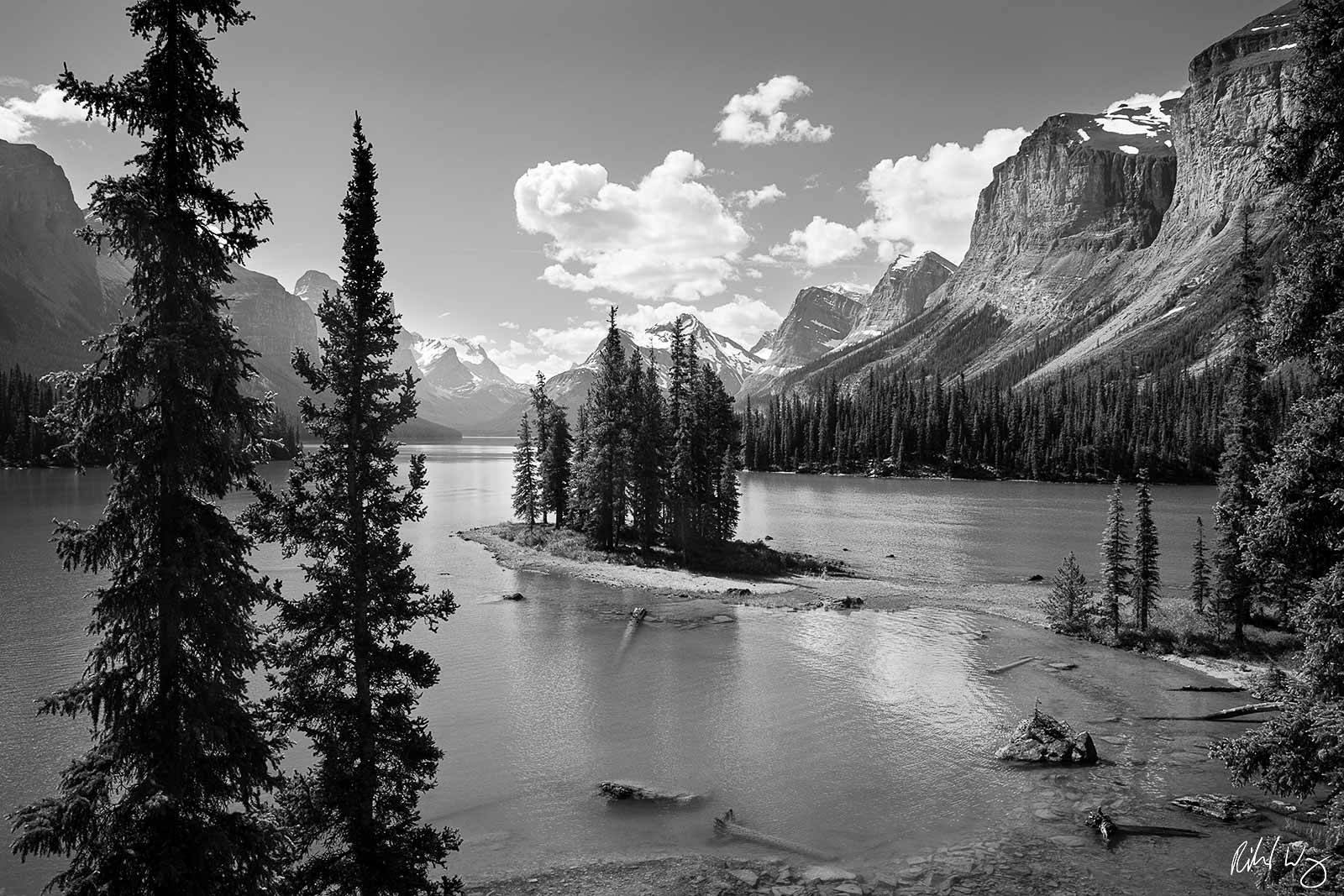This black-and-white photograph captures a serene, natural landscape featuring a lake bordered by dramatic cliffs and mountains with lightly snow-capped peaks in the background. The shoreline is diverse, with a small forested island or sandbar extending into the lake, adorned with a dense collection of trees. The foreground on the left side of the image includes two prominent trees, while the bottom right corner displays a cluttered, dirty shore, possibly the aftermath of a recent storm, with discarded items and driftwood washed up on the sand. The waterway, which reflects the sunlight, extends towards the mountainous backdrop, creating a stunning contrast with the clear sky and scattered clouds. A signature in the bottom right corner suggests the artistic or photographic nature of the image.